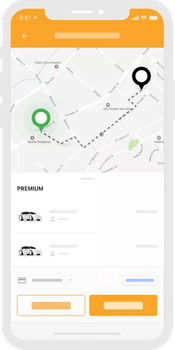**Caption:**

A mobile app screenshot featuring a rideshare interface, resembling those of Uber or Lyft. The screenshot displays a vibrant orange header at the top, with the current time indicated as 9:41. Beneath the header, a map showcases a route depicted by gray dotted lines connecting two points: a green bubble on the left and a black bubble on the right. 

Located below the map, a title labeled 'Premium' appears on the left side, accompanied by two car images resembling sedans. The detailed information next to these cars is obscured, appearing in gray boxes. At the bottom of the screen, there are two buttons. The button on the left is white with an orange outline, while the button on the right is solid orange. The text within both buttons has been redacted, rendered unreadable.